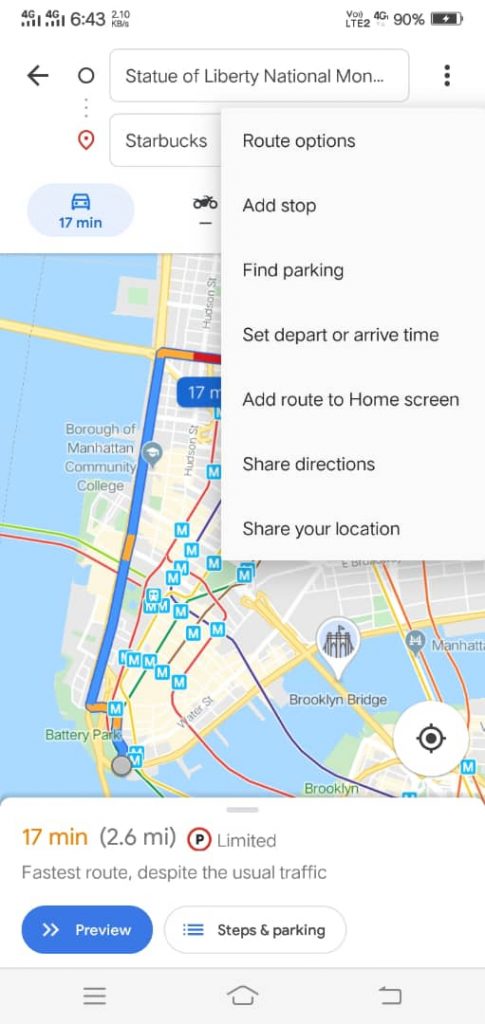This image is a detailed screenshot from a smartphone displaying the navigation interface of Google Maps. The status bar at the top indicates full 4G connectivity with four bars, the current time of 6:43, data usage at 2.10 kilobytes per second, LTE2 network, and a battery level at 90%.

The navigation information details a journey starting at the Statue of Liberty National Monument and ending at a Starbucks location, with a car travel time of 17 minutes. The total distance covered is 2.6 miles. The sidebar on the right side of the screen, shown in a substantial white rectangle, includes several options: 'Route Options,' 'Add Stop,' 'Find Parking,' 'Set Depart or Arrive Time,' 'Add Route to Home Screen,' 'Share Directions,' and 'Share Your Location.' 

Background details on the map display key areas and landmarks such as the Borough of Manhattan Community College, Battery Park, Brooklyn Bridge, and various highways and bridges. Notably, the app highlights that parking is limited and confirms the selected route is the fastest despite usual traffic conditions, also offering the choices to preview the route or view steps and parking details.